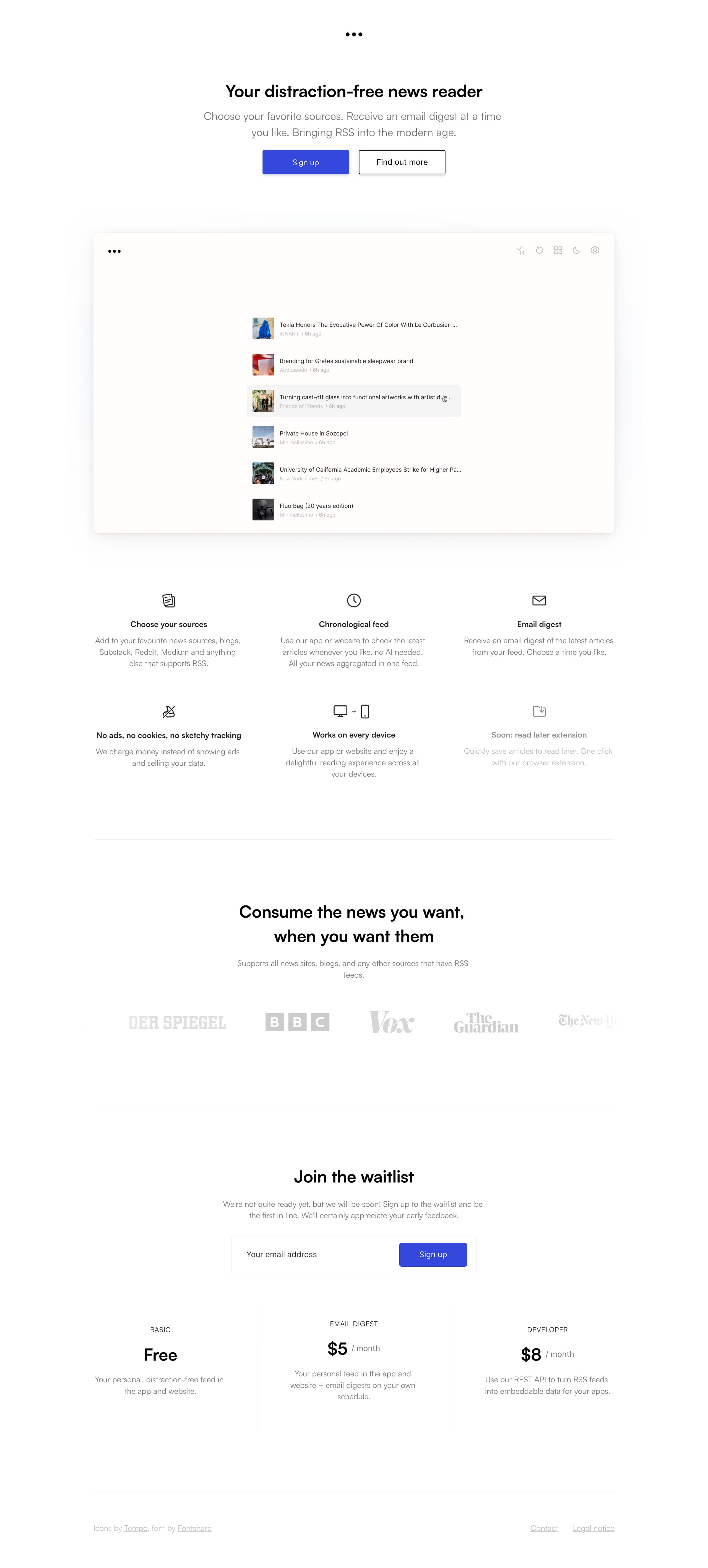Screenshot of a website promoting a distraction-free newsreader service. At the top, a bold tagline reads: "You're a distraction-free newsreader." A subheading elaborates: "Choose your favorite sources, receive an email digest at a time you like, bring RSS into the modern age." Below this, two rectangular buttons provide options to "Sign Up" in blue and "Find Out More."

Underneath the initial information, a large white box displays various article snippets, each indicated by small, hard-to-read text and colorful icons representing different article categories or sources. The timestamps for each article are also visible.

Further down, six distinct blocks describe the service's features:

1. "Choose your sources"
2. "Chronological feed"
3. "Email digest"
4. "No ads, no cookies, no sketchy tracking"
5. "Works on every device"
6. "Soon: Read later extension"

Each block includes a brief explanation of the respective feature. A promotional message below reads, "Consume the news you want when you want," followed by a note that the service "supports all news sites, blogs, and any other sources that have RSS feeds."

At the bottom of the page, there is an invitation to "Join the waitlist," featuring a field to input your email address and a blue "Signup" button. The pricing structure for basic, email digest, and developer plans is also highlighted.